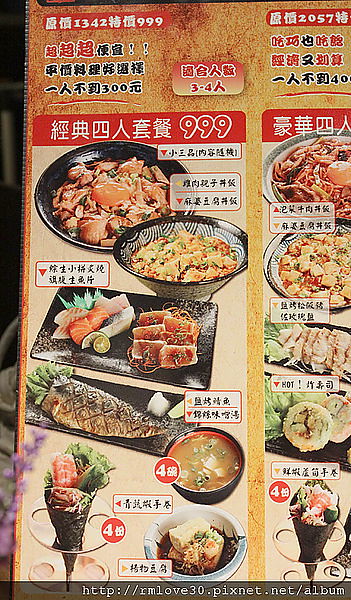The photograph depicts a vibrant, colorful menu, seemingly of Japanese cuisine, with textual details prominently displayed in Japanese characters and punctuated by occasional numeric entries. This menu is divided into two main columns featuring stylized sections with combinations of red and black bars, as well as a variety of vividly presented food items. 

On the left side, a prominent red bar at the top displays the identifier "1342999," leading into a section rich with Japanese characters. Below this, another red bar marked "999" introduces an array of food images. The topmost image shows a black plate with orange-colored meats, possibly chicken or other grilled items, followed by a black bowl adorned with white designs holding noodles. Underneath, slices of fish, which may be sushi or sashimi, are meticulously arranged on a black plate. Further down, another black plate features a whole fried fish, its body marked by crisscross scores. The bottom left displays colorfully contrasting bowls in black and white and a circular glass item containing a black cone stuffed with vegetables. A red circle with the number 4 is also notable in this section.

The right column commences with a red bar displaying "257," and similarly, Japanese characters are intermixed. Below this section are more food images which include multiple white bowls with variations of noodles and a black plate with sliced meats. Further down is a black plate of vegetables and another round glass structure containing a black cone with vegetables peeking out. At the bottom left corner of this side, there's a hint of a purple plant that's out of focus, contributing an element of natural aesthetic.

At the very bottom of the menu, a gray bar reads "http://rmlove3d.pics.net.net.album," serving as a watermark or source link for the image. The back of the menu suggests a colorful, textured canvas, enhancing the vibrant and energetic presentation of the text and images.